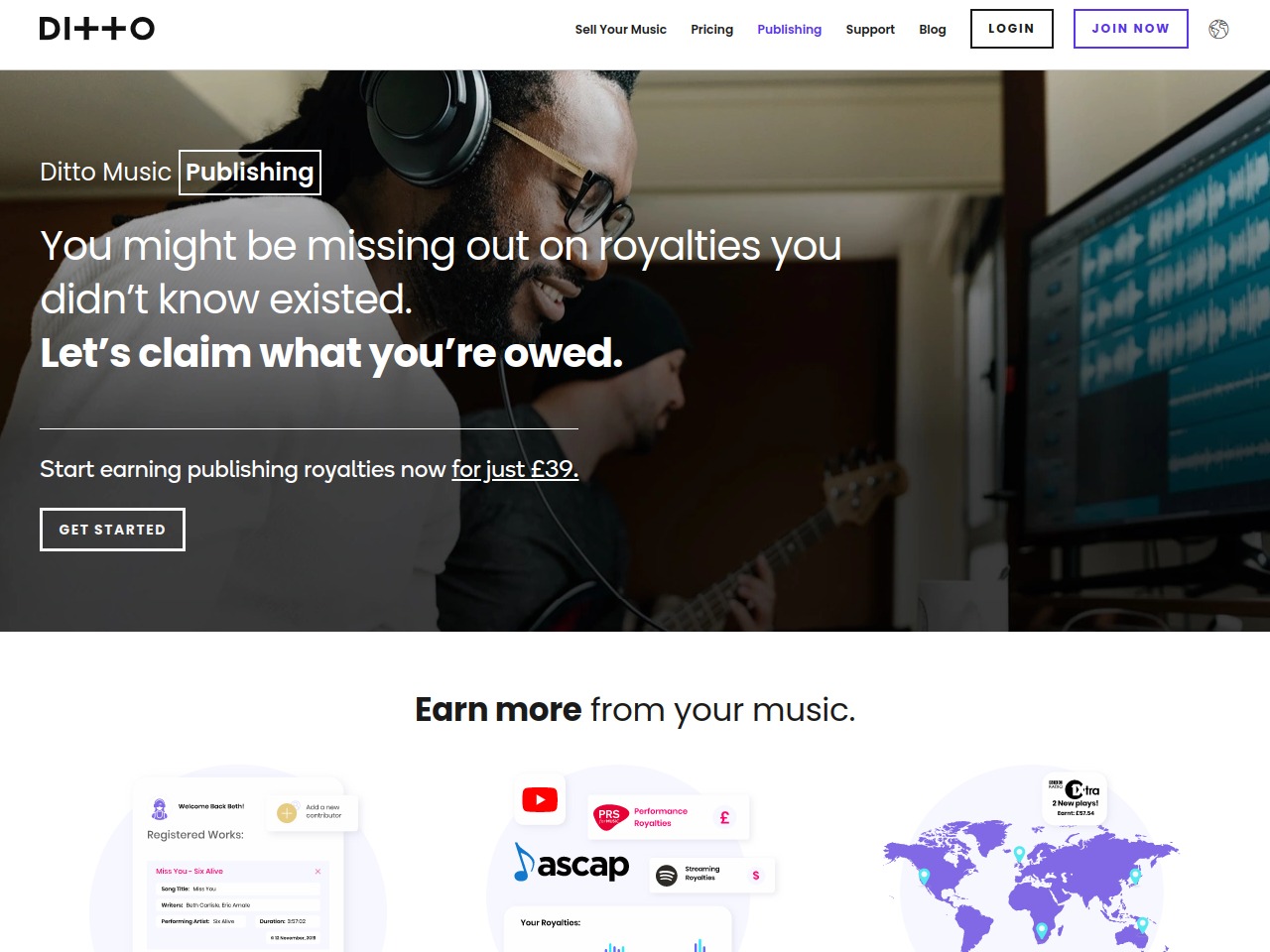This is a detailed screenshot of a promotional page on the Ditto Music Publishing website. In the upper left corner, there is a distinctive logo spelling out "DITTO," with the "T"s styled as crosses in black against a white background. Next to the logo, a navigation menu includes options for "Sell Your Music," "Pricing," and "Publishing" highlighted in purple, followed by "Support," "Blog," and buttons for "Login" and "Join Now."

The main feature of the page is a central image showing a black man with headphones on, dressed in a white shirt, seated in front of a computer screen displaying music software. A Caucasian man wearing a black hat and holding a guitar stands behind him. Superimposed on the image in white text is the message: "Ditto Music Publishing: You might be missing out on royalties you didn’t know existed. Let’s claim what you’re owed. Start earning publishing royalties now for just £39."

Below the image is a prominent "Get Started" button. Beneath this section, a white banner features the text "Earn more from your music" in black, flanked by icons for YouTube, ASCAP (depicted with a blue note), Performance Royalties, Spotify, and other royalty-related symbols.

On the left-hand side, there is a section welcoming returning users with "Welcome Back" and "Registered Works" displayed, though the text in a box below is not readable. The right side of the page features a world map in purple, marked with blue pins that highlight locations in the United Kingdom, the United States, the southern tip of Africa, Australia, and Southeast Asia.